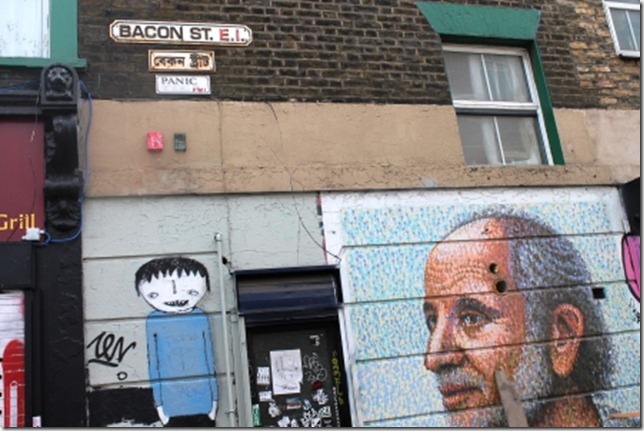This image depicts a large, eclectic building featuring a blend of commercial and residential elements. The ground level appears to be a store, while the upper levels seem to house apartments. The top section of the building is constructed from red brick and boasts a prominent white sign with black lettering that reads "Bacon Street," accented by red "EI" letters. Several smaller signs are present, including one that says "Panic." Below the brick section, the building transitions into a concrete facade adorned with a red box, a gray box, and a green-framed window. Just above the window, a vent is visible. 

Further down, the building features a gray wall that serves as a canvas for urban art. Among these artworks, there's a person painted with a long, exaggerated body, donning a blue shirt, black hair, and a quirky face characterized by a small mouth and prominent teeth. The word "Zen" is inscribed beside the figure. Dominating the side of this wall is a large mural rendered in shades of blue and white, depicting an elderly man with gray hair, a mustache, and a beard. This vivid combination of architectural styles and street art creates a captivating visual narrative.